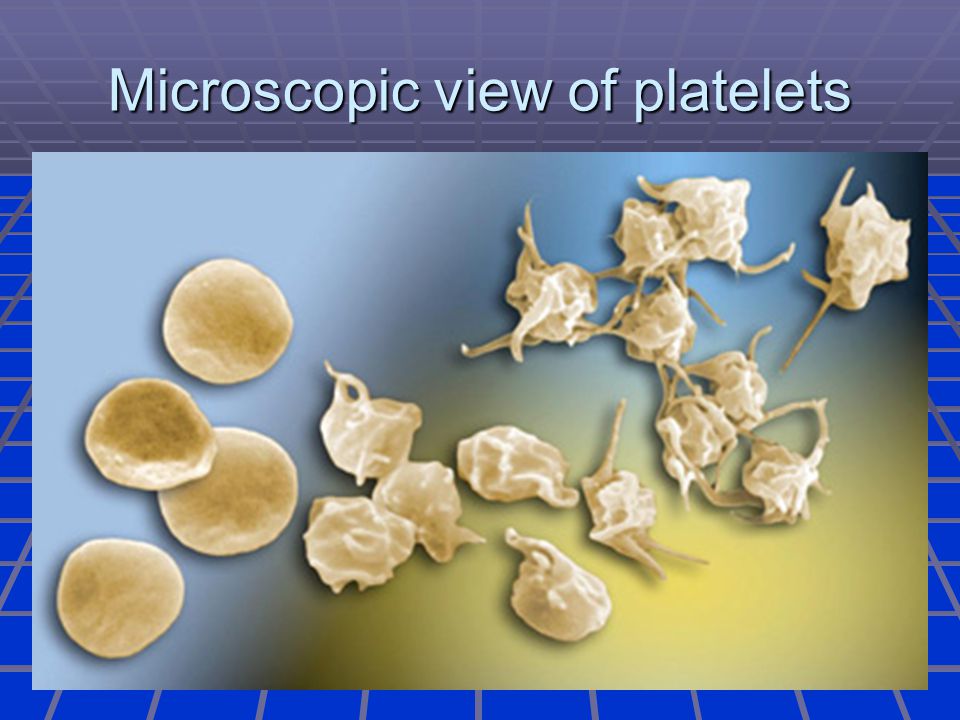The image is an educational presentation slide featuring a zoomed-in, microscopic view of platelets. The slide has a title at the top in light blue font that reads "Microscopic View of Platelets", set against a background displaying a grayish grid pattern that gives a sense of perspective. The main image depicts platelets, predominantly displayed in goldish, whitish, and tan hues with gradient variations. On the left side of the image, four circular, perfectly round platelets are arranged together, while on the right side, the platelets appear more disheveled and irregularly shaped, with tentacle-like extensions. The background of the platelets transitions from a dark gold at the bottom right corner to a black and then to a grayish-blue towards the upper left, reminiscent of a gradient from yellow to blue. Overall, the image has the appearance of being part of a slideshow or screen capture from a slideshow. Additionally, there is a note at the bottom suggesting, "For more information, visit www.FEMA.gov."